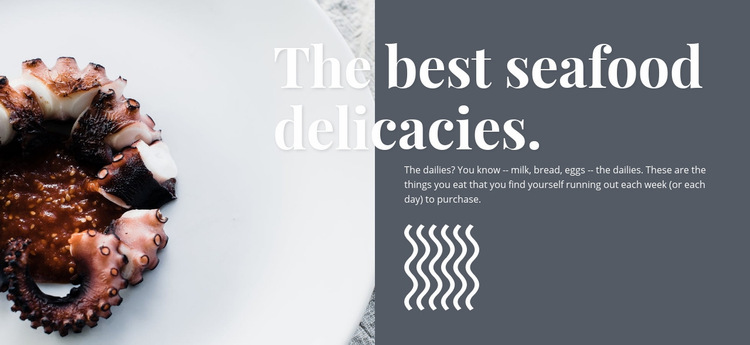The advertisement features a prominently displayed white plate or bowl on the left side. The plate is adorned with a grayish border accented with intricate white etchings along the top and bottom edges. Resting on the plate is a grilled squid, which at first glance might be mistaken for a dessert. The squid is predominantly white, showcasing its tentacles, and has sections that are charred to a darker, almost black, hue from grilling.

On the right side of the advertisement, the background transitions to a blue color. Overlapping the plate and extending into the blue background is the tagline "The Best Seafood Delicacies" written in white. Below this, within the blue section, another text reads "The Dailies: Your daily essentials like milk, bread, and eggs. The Dailies ensure you never run out."

Additionally, the design includes six wavy lines reminiscent of the iconography from Ghostbusters, executed in a similar white and blue color scheme.